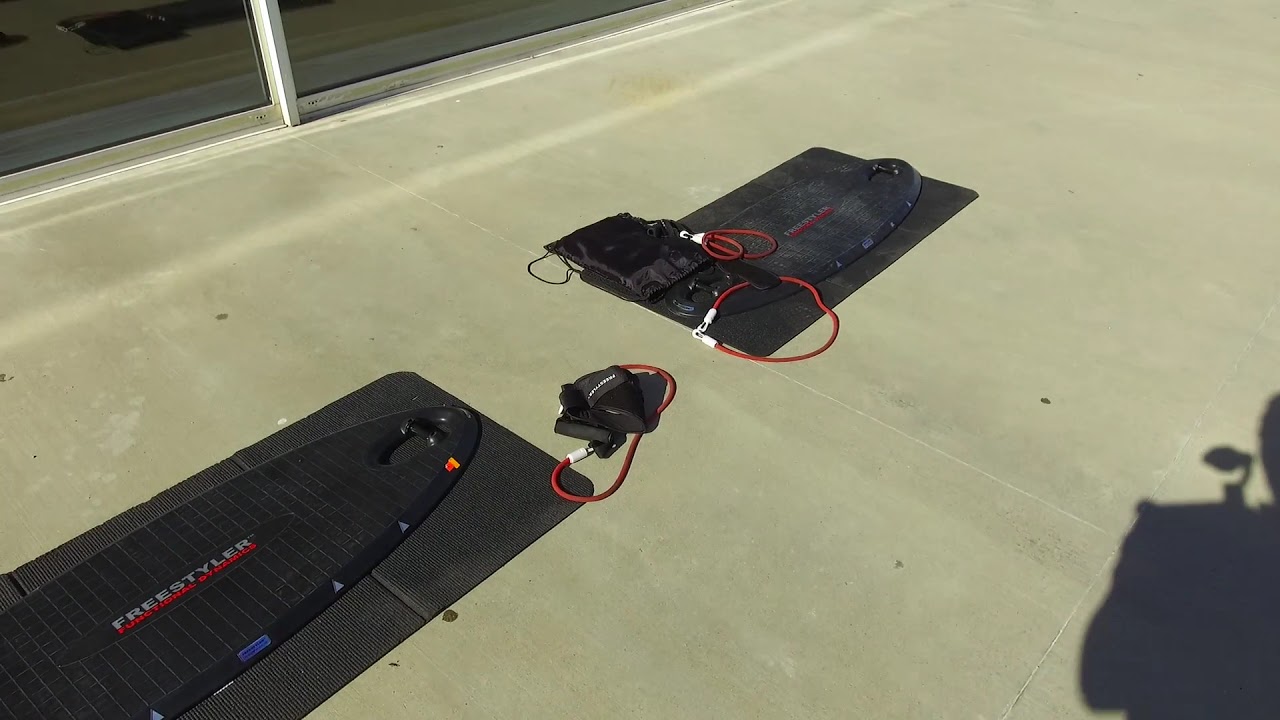In this outdoor photograph, taken on a sunny day, you can see two Freestyler Functional Dynamic boards placed on black rubber mats to protect their bottoms from the concrete ground. Each board is shaped similar to a surfboard and features a handle connected to the board, designed for exercise rather than water sports. The boards are equipped with ankle lines, which are red straps secured with Velcro, intended to keep the boards attached to the user. Additionally, there are small black boxes and electrical wires, one red and one white, potentially part of the exercise equipment setup. The photo also captures a shadow in the lower right-hand corner, likely from the person taking the picture, hinting at their presence and the clear, bright weather.